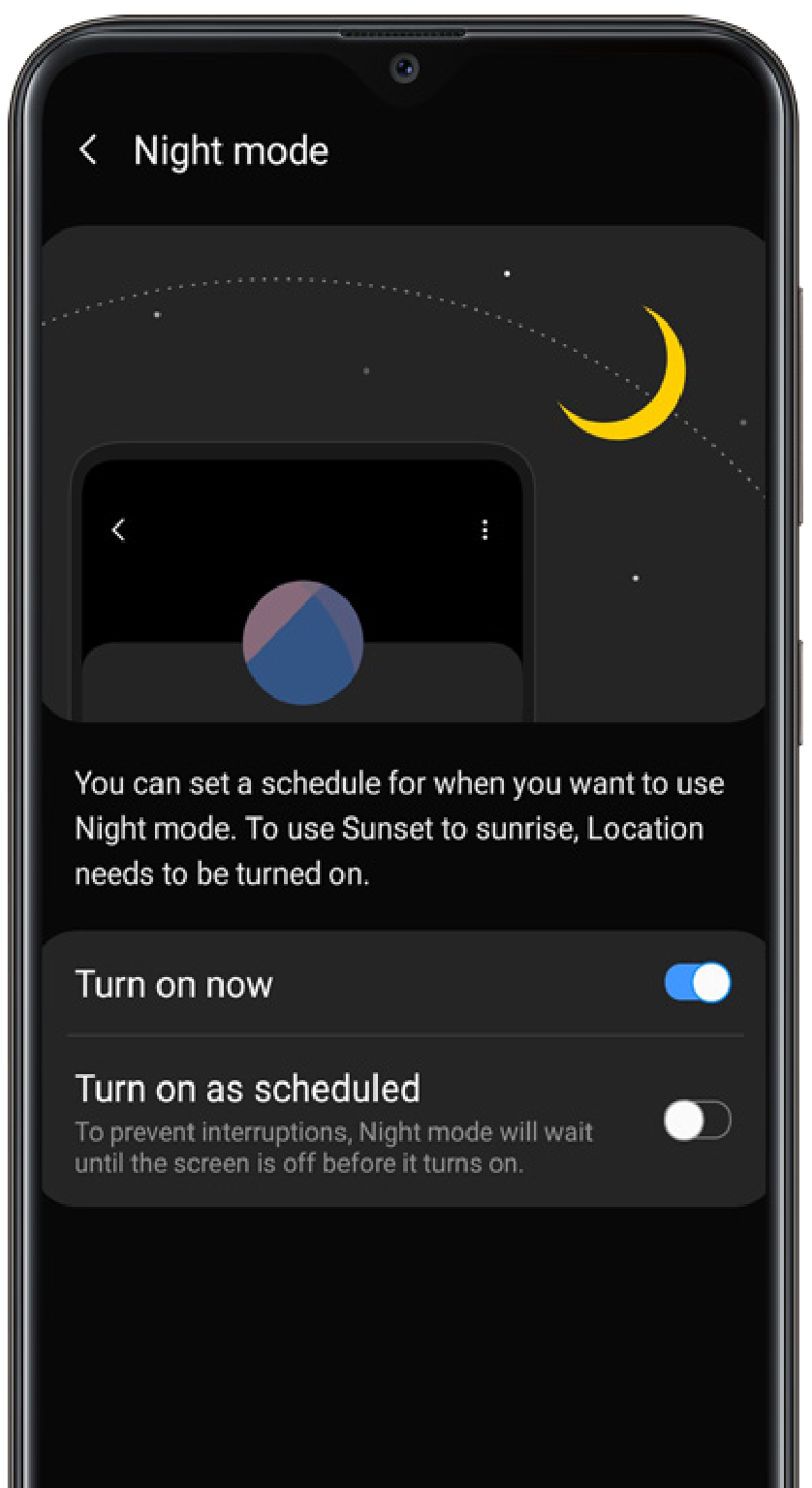This image shows a smartphone screen displaying the Night Mode settings interface. The top of the screen has a black background with "Night Mode" written in white text. To the right of the text, there is an icon of a phone next to a moon. Below this, there is an informational text explaining that you can set a schedule for Night Mode, which activates automatically from sunset to sunrise if the location settings are turned on.

Underneath this information, there are two main sections. The first section features an option labeled "Turn on now," indicated by a blue toggle switch, which is currently in the "on" position. The second section is labeled "Turn on as scheduled," and it is currently turned off. There is also a note explaining that to avoid interruptions, Night Mode will wait until the screen is off before activating.

The overall interface is simple and user-friendly, displaying white text on a dark background along with some star and moon graphics. The phone's brand is indistinguishable, although it appears to resemble an Android device.